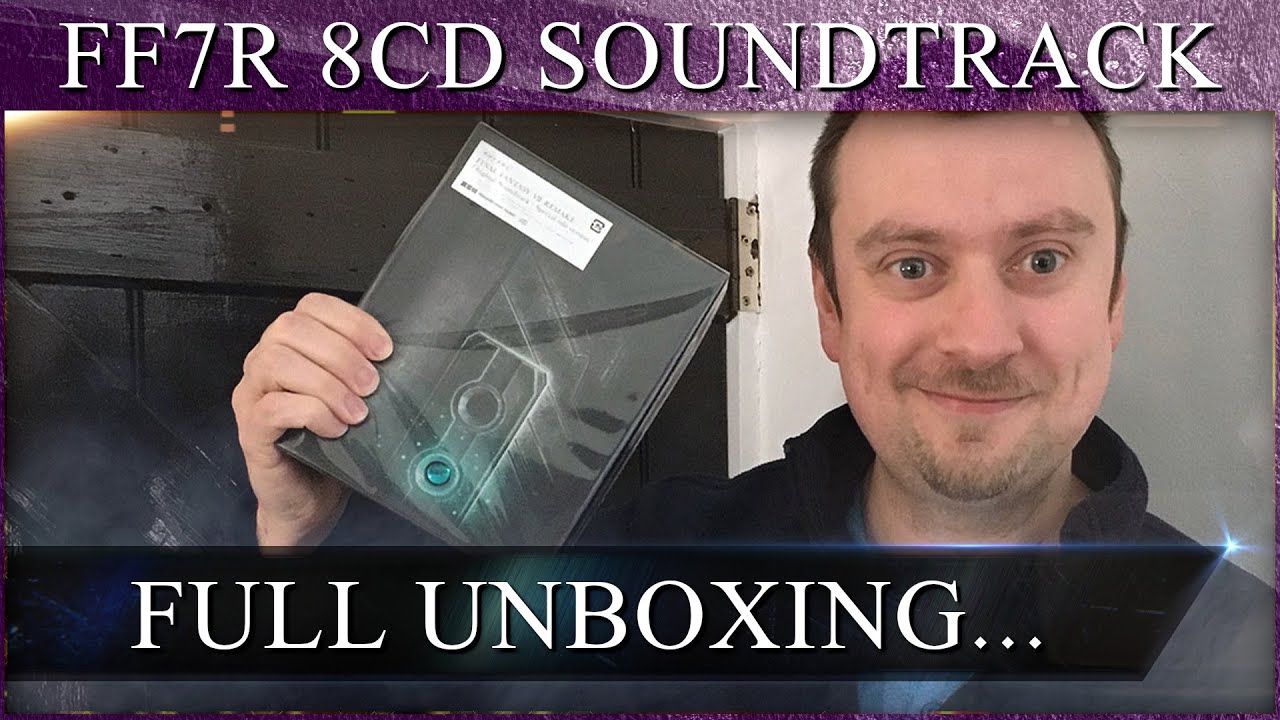The image appears to be a thumbnail for a YouTube video or similar content, featuring a pale Caucasian man with blue eyes, bushy eyebrows, and a receding hairline. He has short hair, a short mustache, and a very short goatee. The man is smiling with a closed mouth and is wearing a mock neck sweater. He stands in front of a white wall and a vintage-looking dark brown door with metal hinges. The most prominent aspect of the image is the man holding a black case with a plastic cover and a visible white label, presumably containing the FF7R 8 CD Soundtrack. At the top of the image, the text "FF7R 8 CD SOUNDTRACK" is displayed in a white font with a black shadow outline on a purple textured background. The bottom of the image features the text "FULL UNBOXING" in bold white font over a mostly opaque black rectangle. The background details, key text elements, and context suggest this is a promotional image for a video unboxing of the soundtrack set.